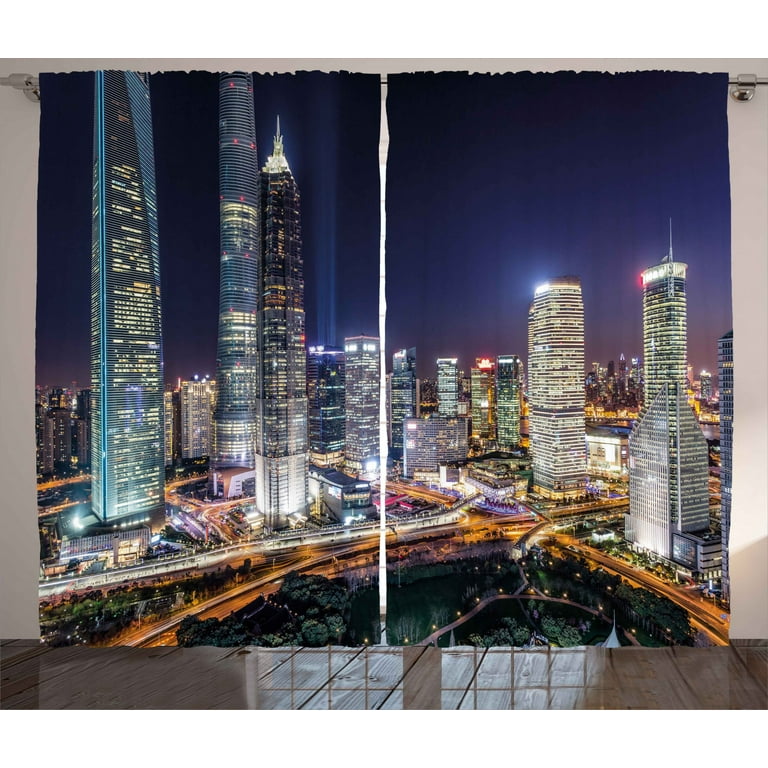The image depicts a set of curtains adorned with a nighttime cityscape photograph showcasing a densely populated urban environment. The curtains feature five prominently illuminated skyscrapers, with three on the left and two on the right, set against a dark blue-black midnight sky. The city is alive with an array of glowing office lights within the buildings and yellow-lit roadways bustling with traffic. There is a park visible at the bottom of the image, and an elevated roadway running above a body of water, reflective of a vibrant city at night. The curtains are held by a metal pole, with a subtle seam in the middle where they meet, and there is a peculiar reflection on the wooden floor, hinting at windows behind the curtains. The entire scene is imbued with the luminous city lights, creating a striking contrast against the dark night sky.